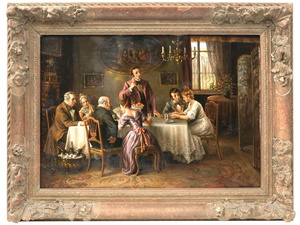This painting depicts an elegant gathering set in what appears to be the late 18th or early 19th century. The artwork features seven individuals—four men and three women—seated around a table, engaging in animated discussion. The women are elegantly styled with intricate updos and wear voluminous dresses characteristic of the era, while the men are clad in formal dress coats. A crystal chandelier hangs overhead, illuminating the scene.

The background of the painting is rich with detail, including several framed pictures adorning the walls. An open window with lavish drapes suggests a connection to the outside world, while a blooming flower on a side table adds a touch of freshness to the setting. A tablecloth covers the main table, where bottles of champagne rest in a chilled bowl, hinting at a celebratory occasion. The room is carpeted with an ornate rug that ties the whole décor together. Additionally, a fireplace adorned with another framed picture above it adds warmth to the composition, creating a painting within a painting.